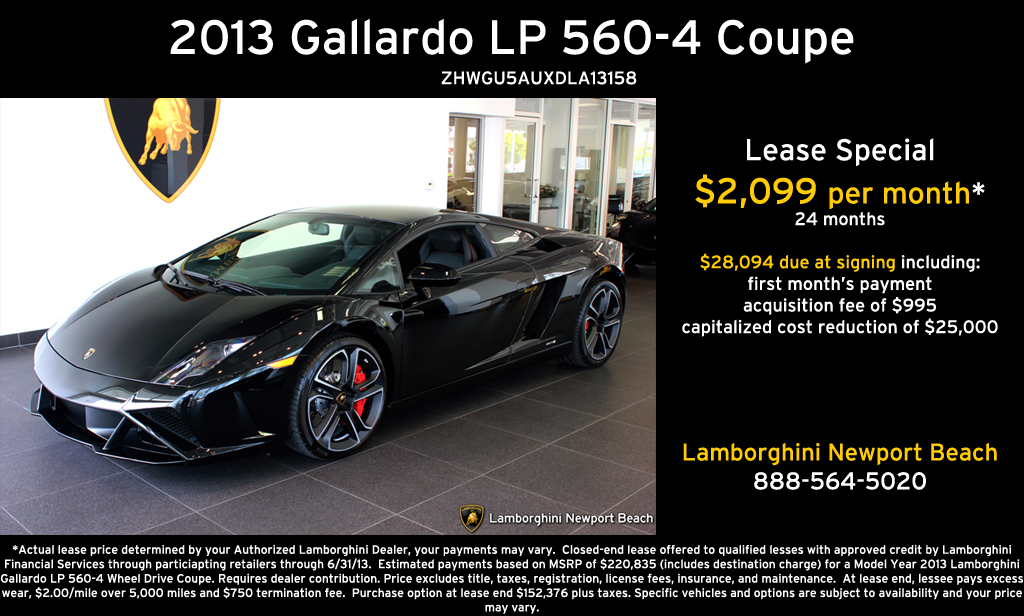This vibrant ad showcases a sleek, black 2013 Lamborghini Gallardo LP 560-4 Coupe, prominently placed slightly to the left and taking up about two-thirds of the image. The car is positioned inside what appears to be a dealership, set against a background of white walls and a tiled floor. Its aerodynamic, two-door design and shiny black rims exude luxury and performance. At the top of the poster, white text clearly states "2013 Gallardo LP 560-4 Coupe" along with a serial number. The right third of the image highlights a lease special, with details outlined as: "Lease Special: $2099 per month for 24 months," "$28,094 due at signing including first month's payment," "Acquisition fee of $995," and "Capitalized cost reduction of $25,000." The bottom-right corner features "Lamborghini Newport Beach" in yellow text with the contact number "888-564-2020" in white below it. A fine print section at the bottom provides further information about the lease terms and conditions.